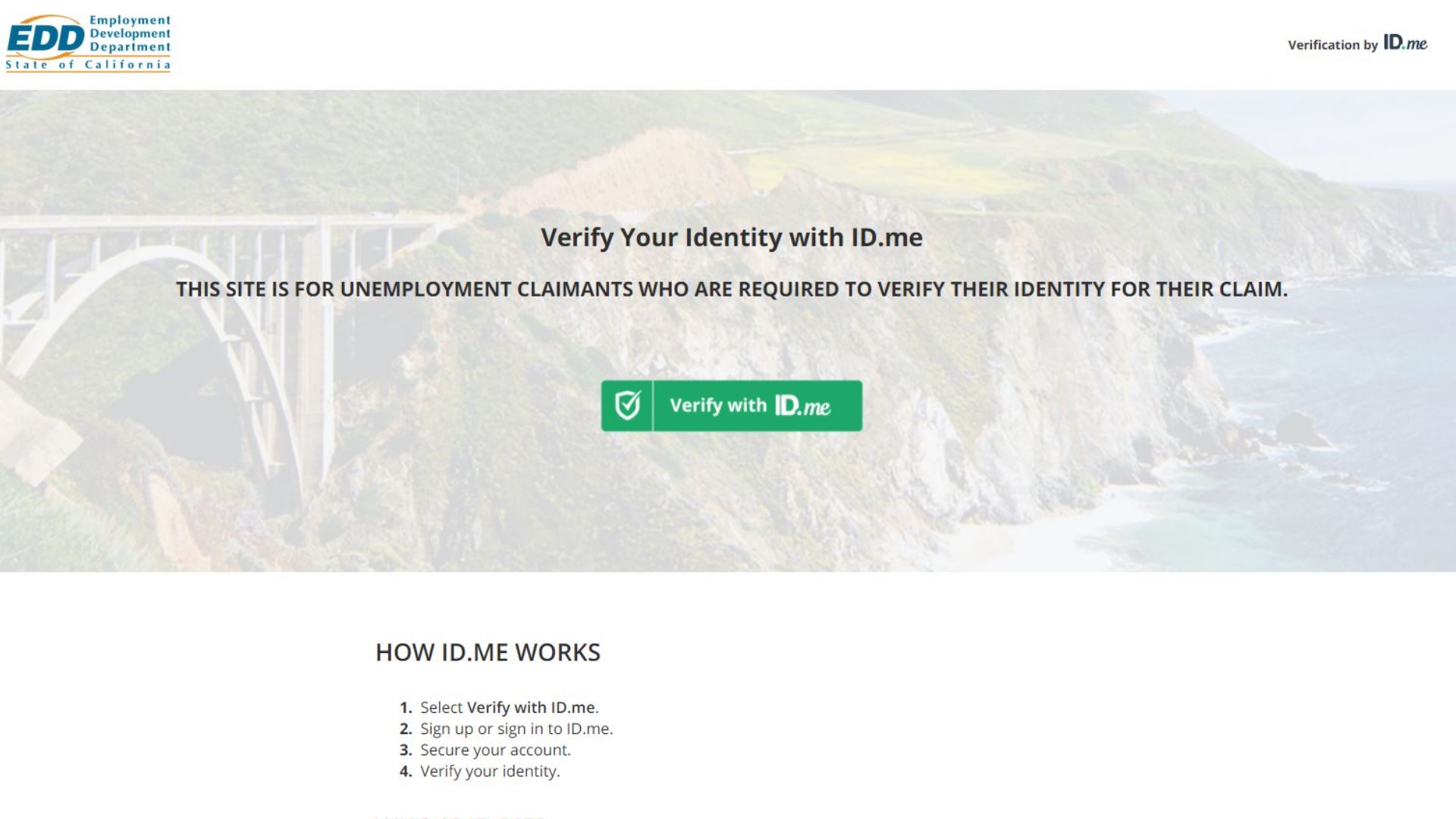A detailed screenshot of the Employment Development Department (EDD) platform. In the upper left-hand corner, the EDD logo is prominently displayed. Below the logo, an image of a picturesque bridge spanning a serene body of water surrounded by mountains sets a serene backdrop. Overlaid on the image is the text, "Verify your identity with ID.me." This page is specifically designed for unemployment claimants who need to verify their identity to proceed with their claims. The site outlines a clear four-step process for verification:
1. Select "Verify with ID.me."
2. Sign up or sign in with ID.me.
3. Secure your account.
4. Verify your identity.
This preliminary screen is an essential step for users to confirm their identity before they can access and use the services provided by the Employment Development Department.